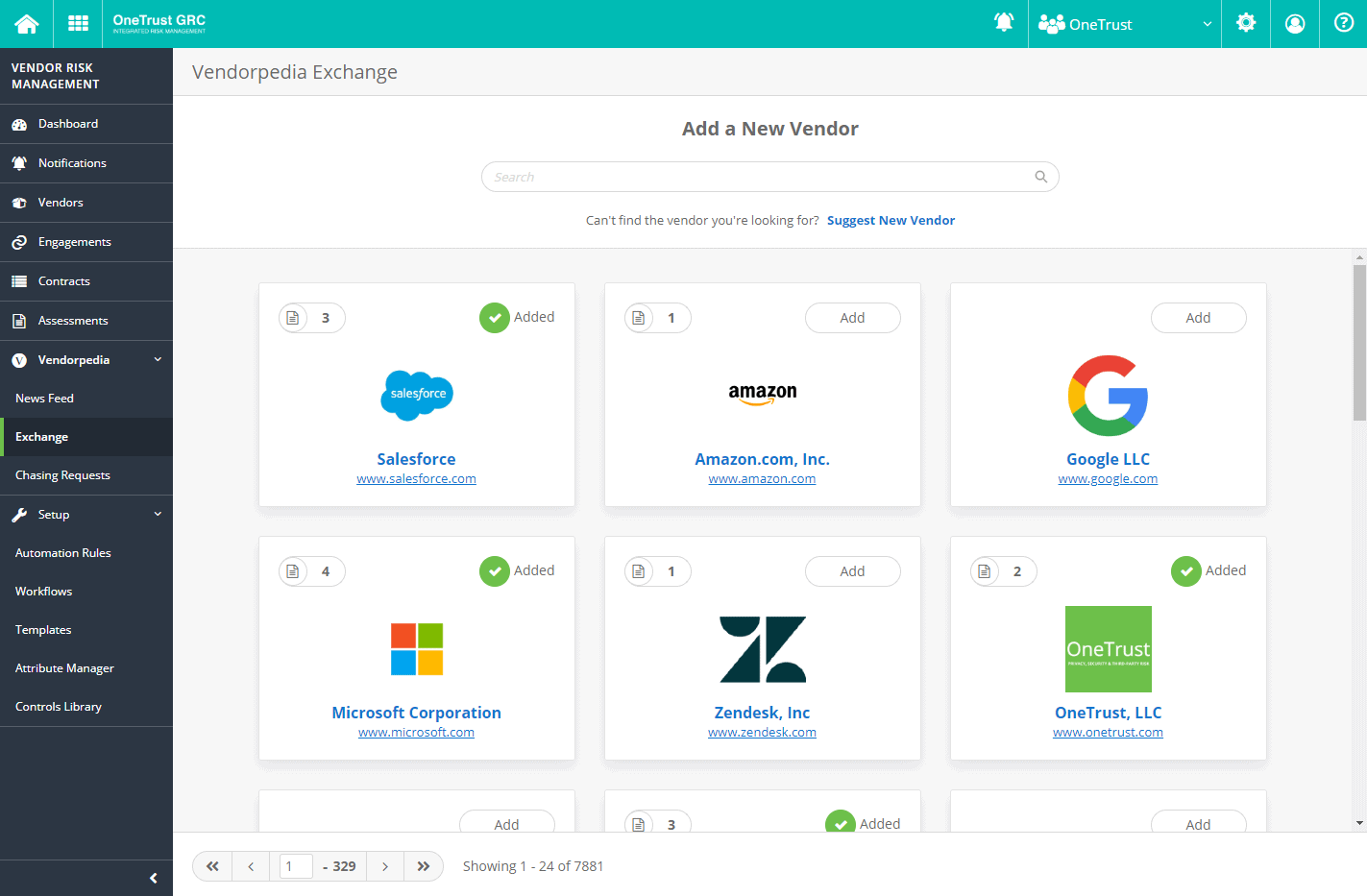The image depicts a user interface for a Vendor Risk Management system. At the top, there is a greenish-blue header bar containing several icons: a house icon, a grid of nine dots, a label "truss GRC," a bell, another label "truss," a downward arrow, settings gear icon, a person icon inside a circle, and a question mark inside a circle.

On the left side, there is a black sidebar with the title "Vendor Risk Management." Below this title are multiple menu items, including dashboard, newsletters, and vendors.

The main section on the right features a "Vendorpedia Exchange" label in a blue box. Below it is a white box with the options to "Add a New Vendor" and a search box. Additionally, there is some blue text, though its content is not specified.

The primary content area has a blue background with six white rectangular cards arranged vertically. Each card has various details:
  
1. **First Card:** 
   - Top label: gray piece of paper icon with a checkmark and the number 3
   - Content: a green circle with a checkmark labeled "Added," followed by a blue cloud icon and the word "Salesforce"

2. **Second Card:** 
   - Top label: gray piece of paper icon with a checkmark and the number 1
   - Content: white "Add" button, followed by "Amazon" and "amazon.com Incorporated"

3. **Third Card:** 
   - Top label: gray piece of paper icon with a checkmark and the number 4
   - Content: green circle with a checkmark labeled "Added," followed by "Microsoft Corporation"

4. **Fourth Card:** 
   - Top label: gray piece of paper icon with a checkmark and the number 1
   - Content: white "Add" button, followed by "Zendesk Incorporation"

5. **Fifth Card:**
   - Top label: gray piece of paper icon with a checkmark and the number 2
   - Content: green circle with a checkmark labeled "Added," followed by "OneTrust LLC"

A slider button is visible on the side to scroll through additional vendors. The view cuts off three more cards indicated to be beyond the initial view.

At the bottom, pagination controls are present: 
   - Double left arrow, single left arrow, number 1, text "-329," single right arrow, double right arrow
   - Label indicating "Sharing 1-24 of however many"

This thorough layout helps users manage various vendors and their corresponding statuses and actions efficiently.